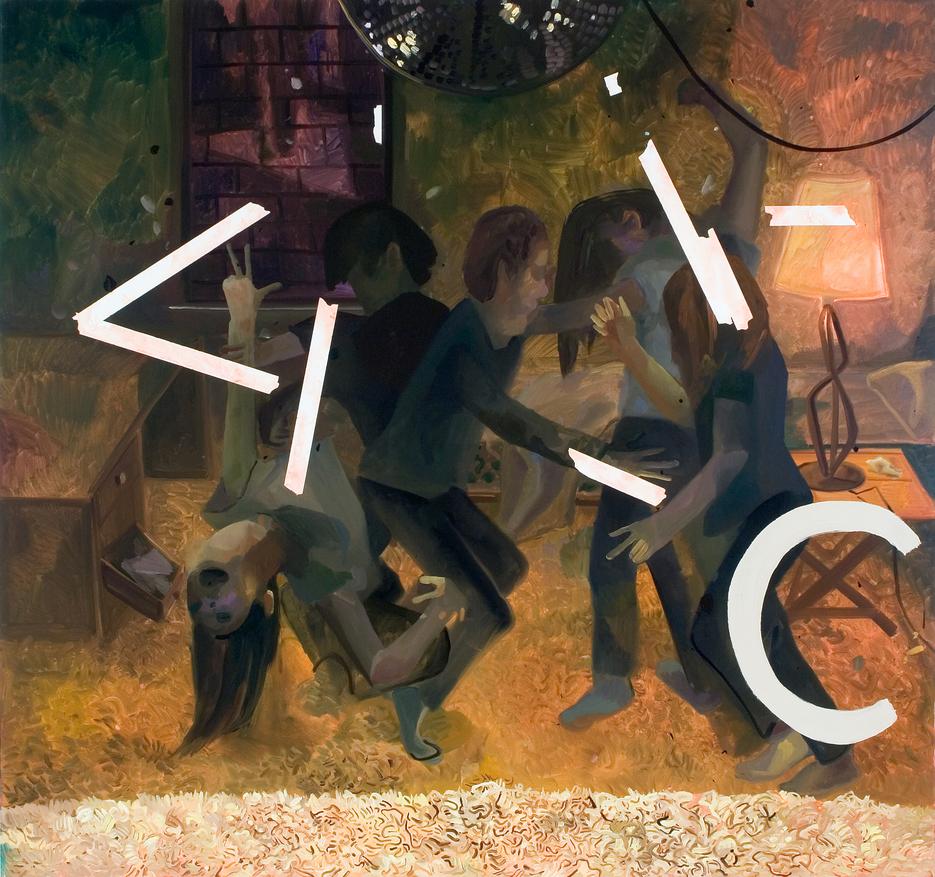The abstract painting prominently features several white markings: a less-than sign (<), multiple slashes (/ and \), two dashes (--), and a letter 'C'. These white marks overlay a scene with five individuals engaged in dynamic motion, portraying either a dance or a struggle. One woman with long hair appears to be falling to the ground while looking up, a couple with reddish hair is dancing together, and another man and woman in the background are engaged in unclear activities. The figures have a 3D, Pixar-like cartoon appearance and all wear blue shoes. The background contains elements such as a lit lamp, a wall resembling stone, and a table with a drawer to the left. The image is rich with colors, primarily blue, brown, orange, green, and purple, giving it a vibrant yet somewhat chaotic feel.